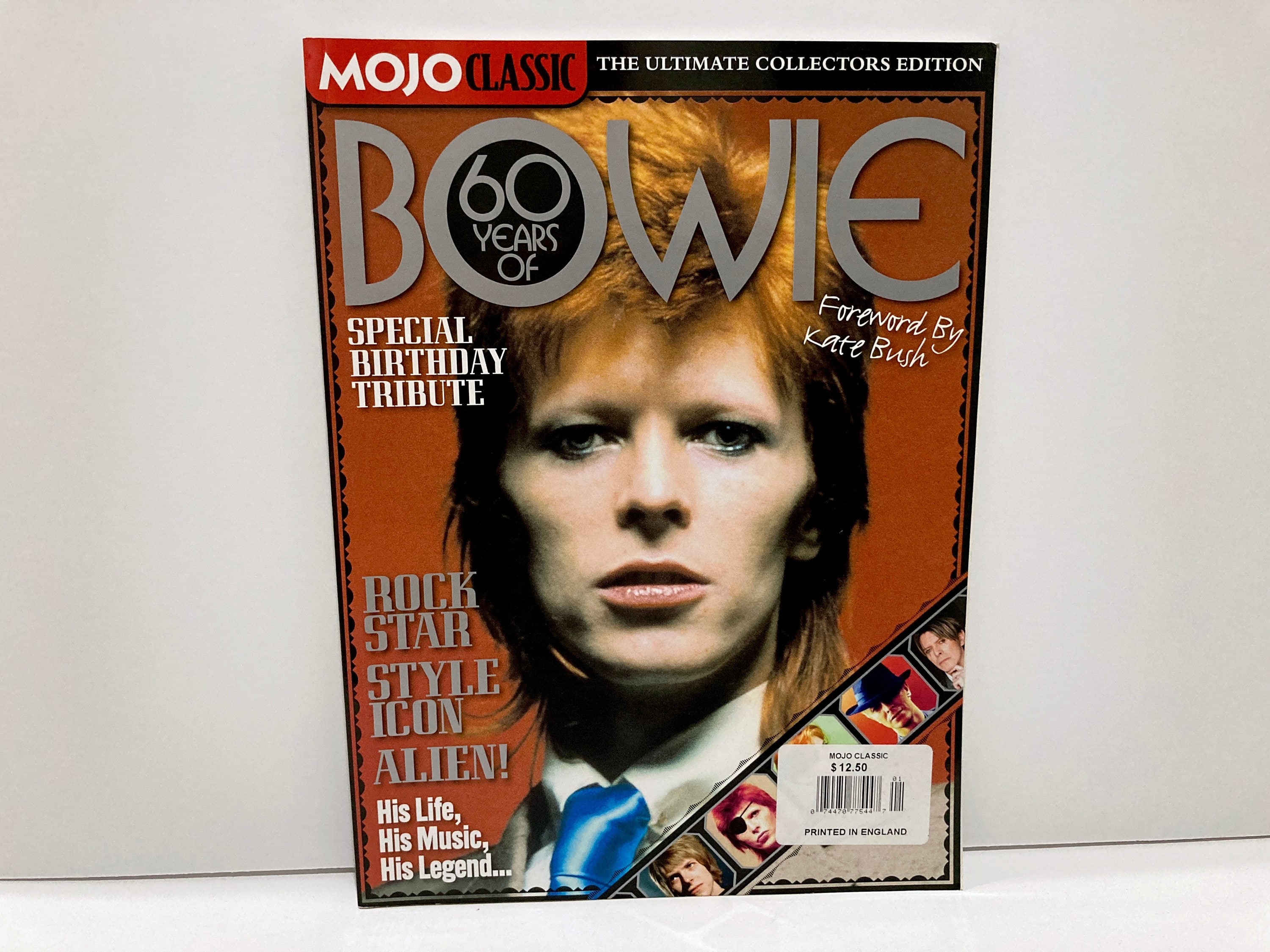This is a cover of a special magazine edition titled "Mojo Classic: The Ultimate Collector's Edition." The cover features a young David Bowie with his pale complexion, reddish spiked hair, and a blue tie over a white collared shirt. The background radiates a burgundy and orangey tint. At the top, a red banner with white letters spells out "Mojo," followed by "Classic" in black. Adjacent to it, a black banner displays "The Ultimate Collector's Edition" in all caps and white font.

The centerpiece of the cover is the phrase "60 YEARS OF BOWIE," where "60 YEARS OF" is embedded inside the 'O' of "BOWIE." Directly beneath, in white text, it states "Special Birthday Tribute." To the right, it mentions "Forward by Kate Bush."

The lower left corner lists some of Bowie's iconic roles in gray text: "Rockstar, Style Icon, Alien." Below that, it reads in white, "His Life, His Music, His Legend." The lower right corner features a price tag indicating "$12.50," and a diagonal strip resembling a photo booth film strip showcases various images of Bowie over the years.